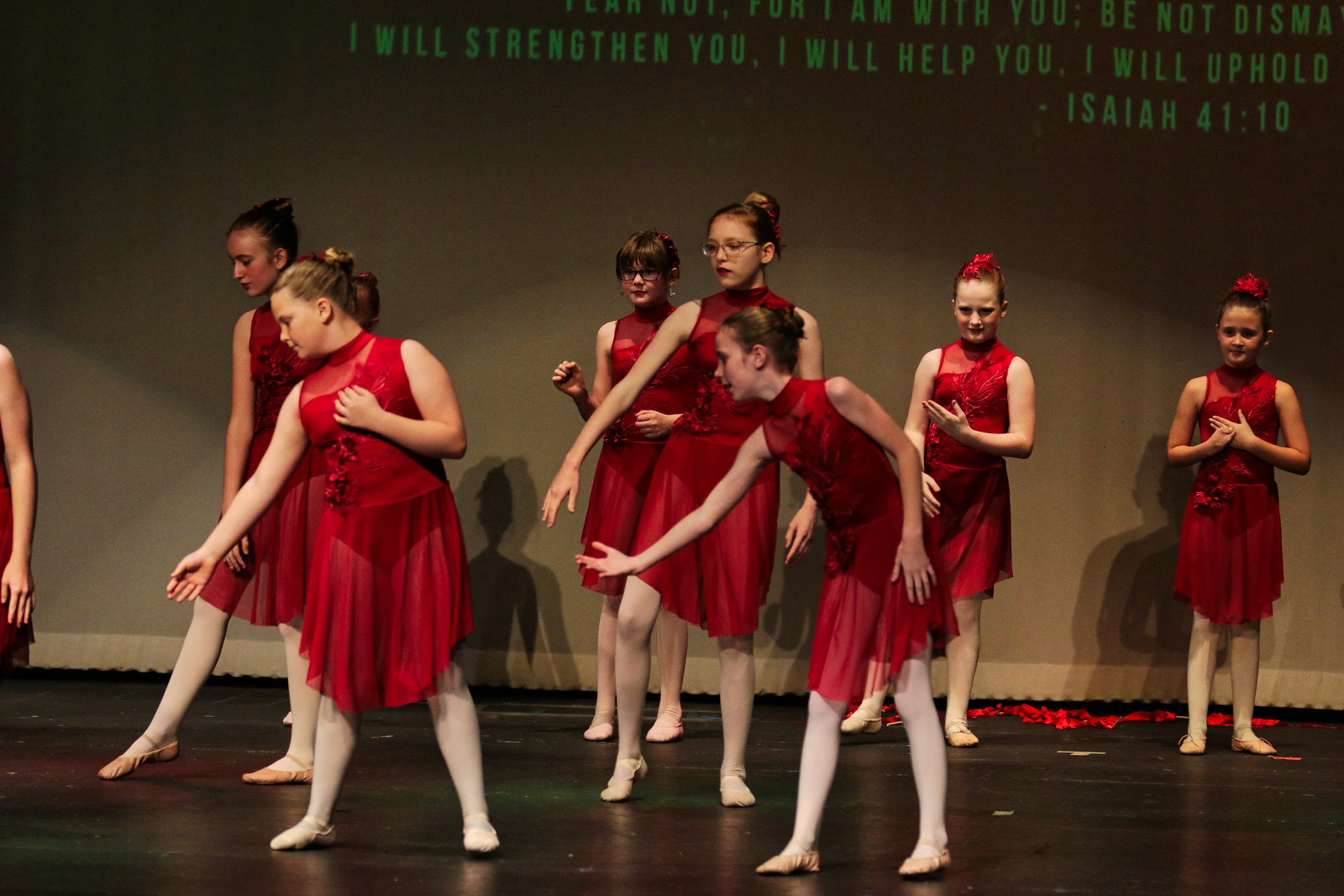This photograph captures a group of approximately seven young girls, likely aged between 10 to 12 years, performing on a stage during a dance recital. They are dressed in matching red dresses that feature tank tops with crew necks and flowy skirts that reach their knees. Each girl wears white tights and pink ballerina slippers, and their hair is styled in buns adorned with red decorative bows. The stage has a black backdrop and hardwood flooring. In the background, there's a Bible verse painted in green text on the wall, with the visible portion reading, "I will strengthen you, I will help you, I will uphold," followed by "Isaiah 41:10." Additional stage decorations include red ribbons scattered on the ground. The overall color palette of the scene includes dark brown, gray, white, red, and green, and the setting appears to be indoors. The dancers are predominantly positioned in the center of the image, with some girls in the front visibly in motion, while those in the back appear to be standing still.